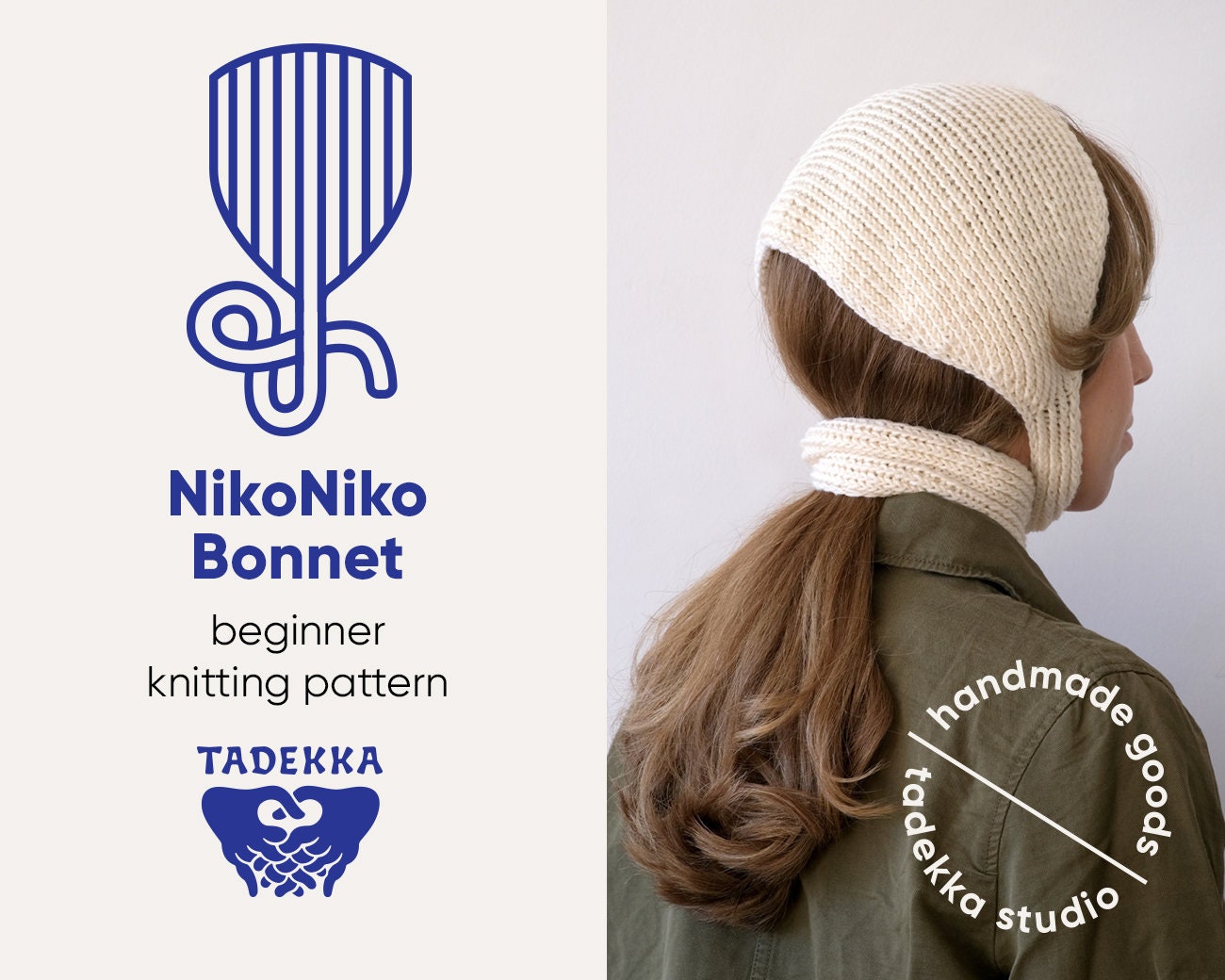The image showcases an advertisement for the "Nico Nico Bonnet" beginner knitting pattern by Tadeka Studio. The left segment of the picture features a detailed drawn illustration of the bonnet, set against a white background. Below the illustration, in blue font, it reads "Nico Nico Bonnet," followed by "beginner knitting pattern" in black font. Further down, in blue, it says "Tadeka" accompanied by a logo depicting two hands clasped together in an interwoven pattern. On the right side, the photo displays a woman wearing the actual bonnet. She has long, dark hair tied in a ponytail and is seen facing away from the camera. She is wearing a white knitted bonnet that covers her head and ears, extends under her chin, and wraps around her neck. She is dressed in an army green jacket and is positioned against a white wall. In the lower right corner of this segment, it says "handmade goods" in a circular font surrounding the phrase "Tadeka Studio."